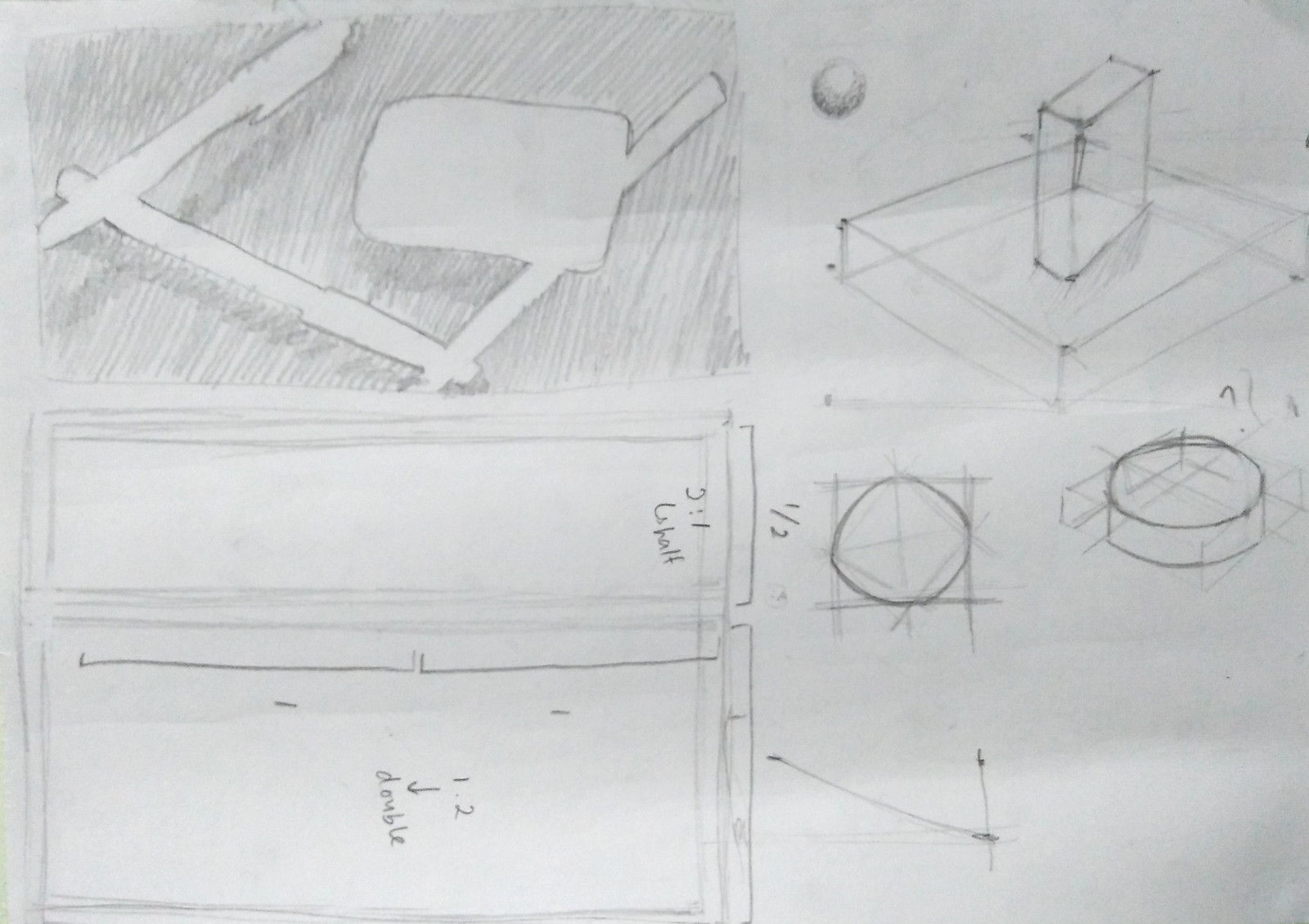In this horizontally elongated, rectangular pencil sketch, various geometric and three-dimensional shapes are meticulously drawn. Starting from the top left corner, there is a shaded quadrant featuring three horizontally aligned pens stacked on top of one another, forming three sides of a square. The center of this area remains unshaded, creating a rectangular cutout. 

In the lower right section of the image, another diagram presents two narrow rectangles placed vertically, one above the other. Handwritten inscriptions nearby include the numeral "1.2" and the word "double," positioned on the lower right side of this particular section.

Moving to the right side of the image, a three-dimensional, cube-like, low-lying shelf is depicted in a perfect square, with a smaller, upward-extending rectangle inside it, also rendered in three-dimensional pencil sketching. Beneath this form are two three-dimensional round objects, adding depth and complexity to the drawing.